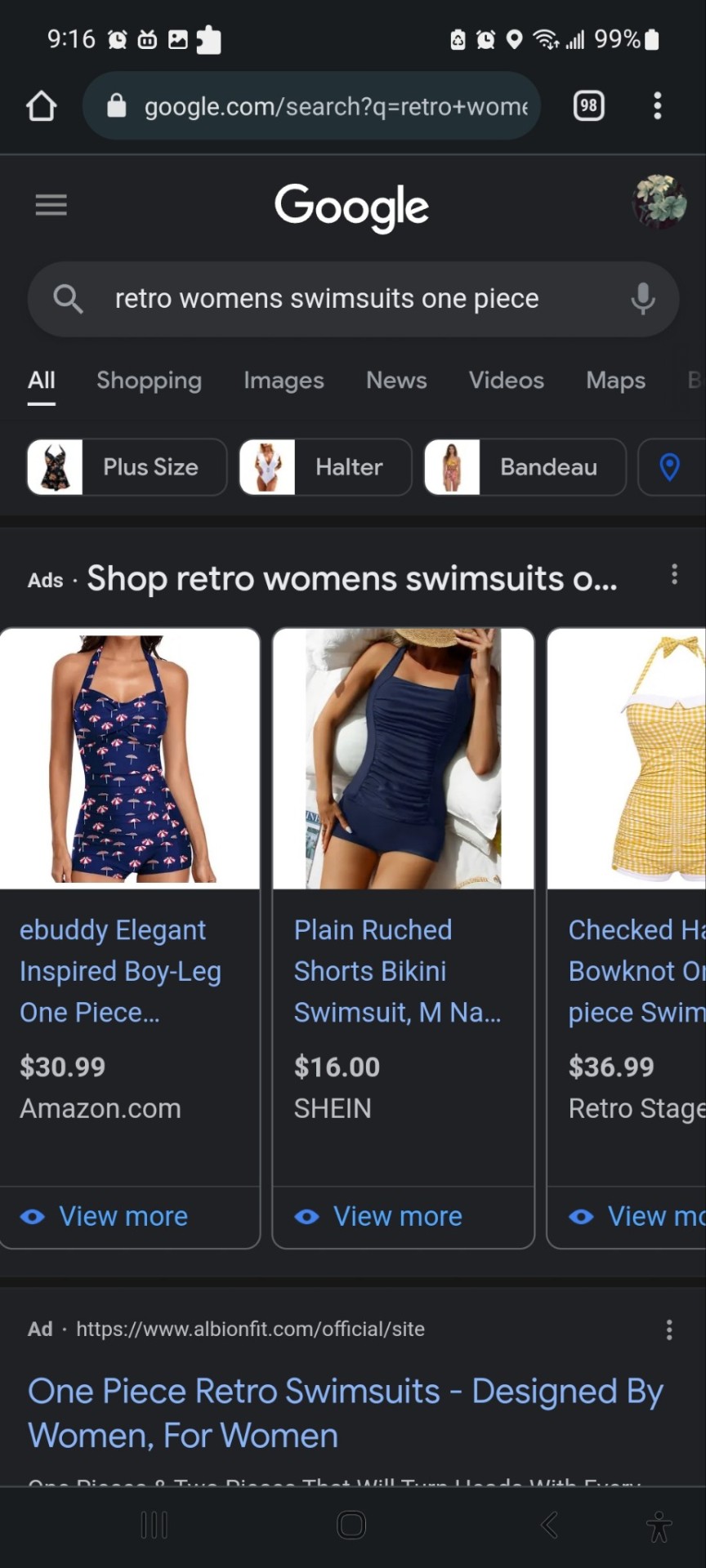This image captures a screenshot of a Google search conducted on a mobile phone for "retro women's swimsuits one piece." The screen features Google's standard search options including "All," "Shopping," "Images," "News," "Videos," and "Maps" at the top. Below these options, clickable filter suggestions like "plus size," "halter," "band," and "bandeau" are displayed. As the user scrolls down, the search results include a selection of one-piece swimsuits for purchase.

The first item listed is an "eBuddy Elegant Inspired Boy Leg One Piece Swimsuit," highlighted by a vibrant royal blue or navy blue color adorned with umbrella prints. Another product listed is a "Plain Ruched Shorts Bikini Swimsuit" available in size medium and also in navy blue. Additionally, there's a “Checkered Halter Bow Knot One Piece Swimsuit," which is shown in a picture without a model.

At the very bottom of the search results, an actionable blue link reads "One Piece Retro Swimsuits Designed by Women for Women," offering users the opportunity to explore further.